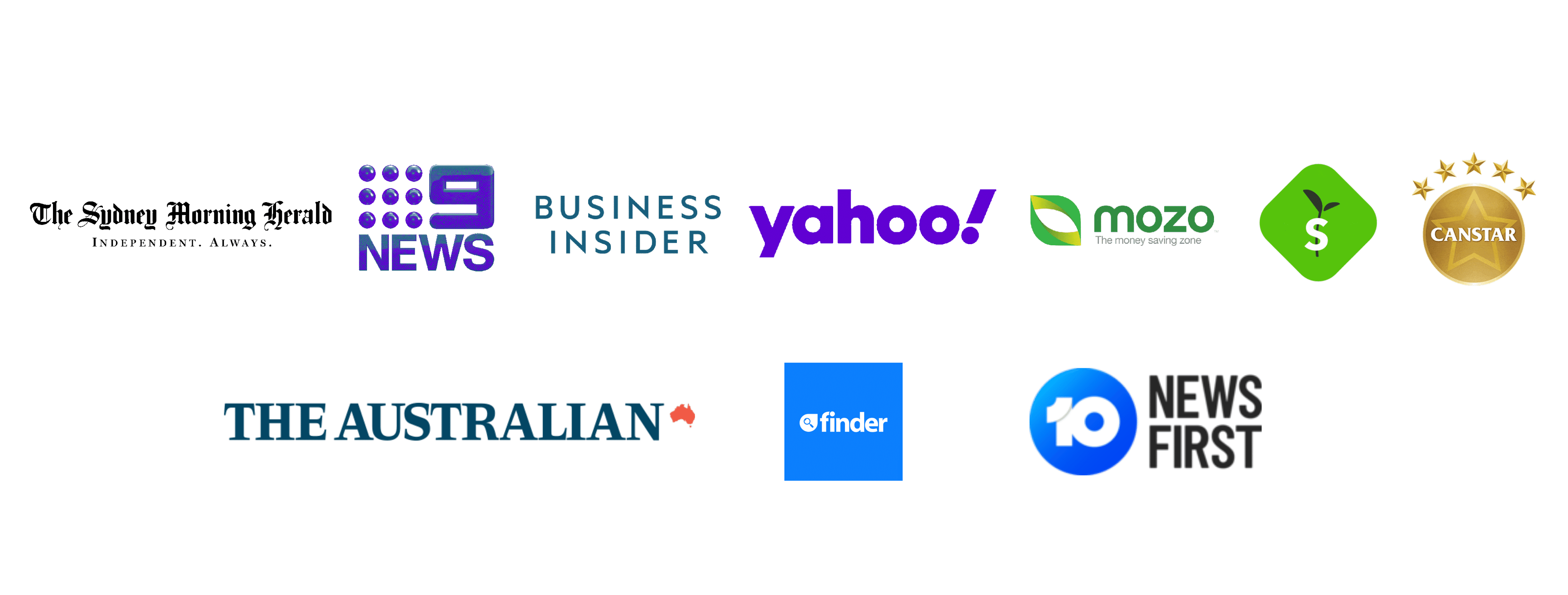A collage of various logos is displayed on a white background, organized into two rows. The top row features seven logos, while the bottom row has three.

In the top left corner is the logo for The Sydney Morning Herald, presented in a font resembling that of The New York Times. Next to it is the 9 News logo, characterized by blue text and nine dots forming the number 9 with "news" written below it. The third logo belongs to Business Insider, depicted in simple blue text. Following that is the Yahoo logo featuring purple text and a noticeable slanted purple exclamation point. The Mozo logo is next, showcasing a green, leaf-shaped design with a white cutout in the center and the word "Mozo" written in green above some unreadable text. To the right of Mozo is a diamond-shaped logo with rounded corners in bright lime green, displaying a black sprig or bud with a white "S" in the middle. The CanStar logo comes next, featuring a gold seal with a lighter gold star and white text that reads "CanStar," circled by five stars forming an arc.

The bottom row starts in the left-hand corner with The Australian logo, followed by a small red silhouette of Australia. Next to it is the Finder logo, which features a blue square with white text and a teardrop-shaped design pointing upwards and to the right; inside the teardrop is a white magnifying glass with a blue lens. Finally, there is a circular blue logo with a white number 10 and the word "News" below it, followed by the text "First" in black.